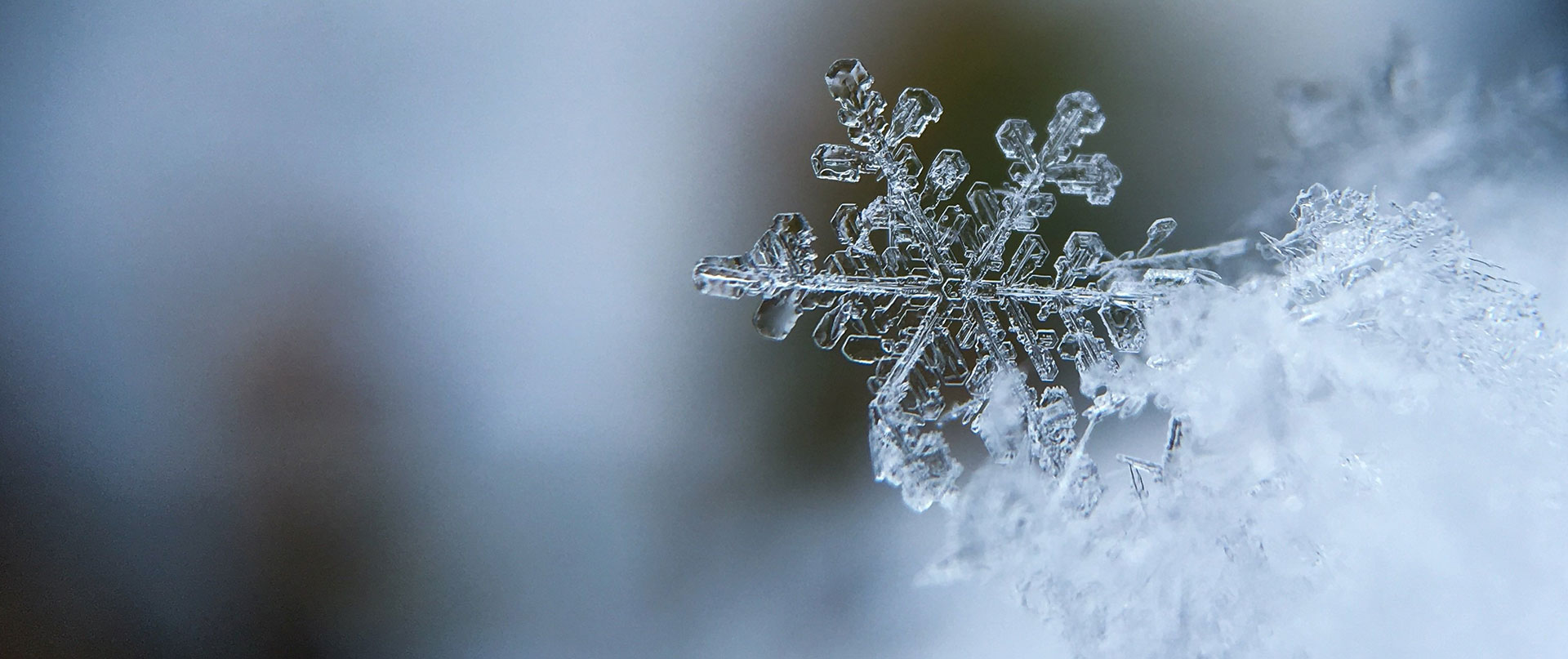The photograph is an extreme close-up image of a single, six-sided snowflake, showcasing its intricate crystalline structure. The snowflake is centered in the frame, with three of its arms very clearly defined, while the other three show signs of melting. It has a delicate, glass-like appearance, indicating it's a real ice formation. The background is softly blurred, with a mix of bluish-white tones and a darker area right behind the snowflake, enhancing its visibility. To the right side of the image, some melting ice crystals can be seen, with additional individual snowflakes attached to them. The overall effect highlights the snowflake's geometric precision and slight moistness, making it stand out against the out-of-focus backdrop.